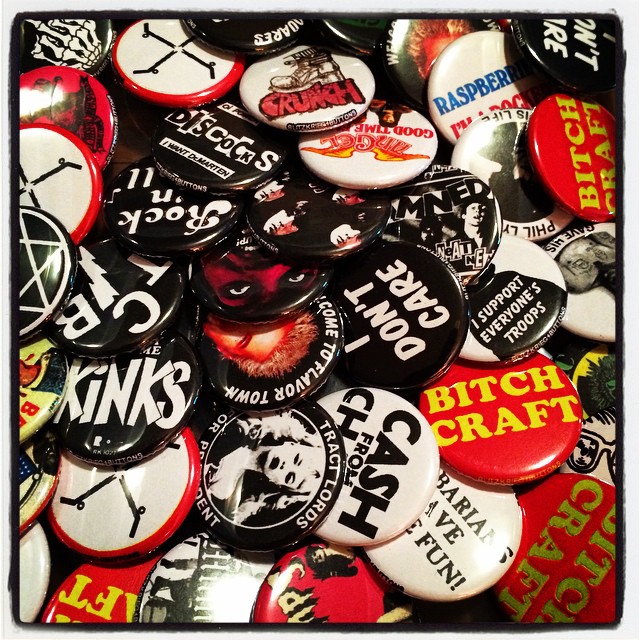The image showcases a scattered assortment of assorted pins and buttons, each with unique messages and designs. The majority of the pins are black, white, or red, with a few featuring yellow text. Many of the pins are oriented facing us, ensuring their messages and images are clearly visible. Among the standout buttons, there are several with the phrase "BITCHCRAFT" in red with yellow text. In the top right corner, notable buttons include one with the letters "N, T" followed by "RE" below, and another black pin with "RASPBERRY" where the letters "RY" are cut off. Additional pins display an array of themes, from punk rock references, such as "The Kinks" and "I Support Everyone's Troops," to various text and images, including depictions of women and faces. The whole collection looks as though it has been casually thrown together, resembling a drawer or a collector's scattered assortment.